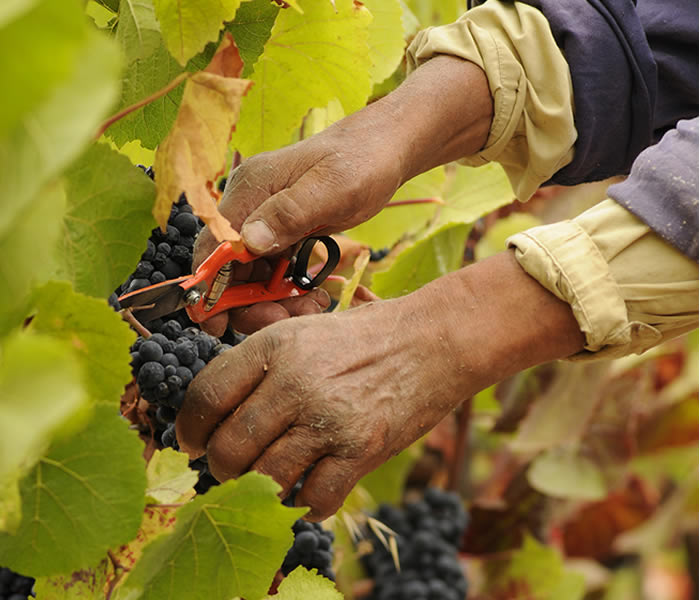The image depicts a close-up of the weathered hands of a laborer engaged in harvesting dark, blackish-purple grapes from vines in a field. The person's hands are rough, worn, and suggest a life of hard physical labor. Clad in a blue shirt over a beige one, both with rolled-up sleeves, the worker delicately maneuvers silver, orange, and black shears to clip grape clusters surrounded by bright green leaves. The warm autumnal colors indicate it's harvest season, creating a vivid contrast with the deep hues of the small grapes, likely intended for winemaking. The photograph captures the essence of meticulous manual labor and dedication to the craft.